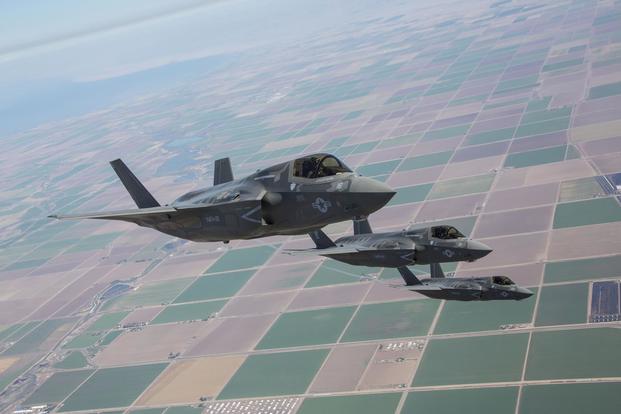The photograph captures a trio of green military fighter jets, each marked with a white cross on the right side front, flying in a diagonal formation over a patchwork of farmland. The farmland below, divided into precise square grids, showcases various hues of green, brown, and yellow, indicating different crop types. The jets, characterized by their pointy noses and twin vertical tail fins, seem to be partaking in training exercises. The aircraft are equally spaced, with the closest one positioned in the bottom left of the image, and the others following diagonally to the right. To the top left, a hazy blue sky is visible, possibly hinting at a nearby water body, highlighting the overall clear, sunny day.